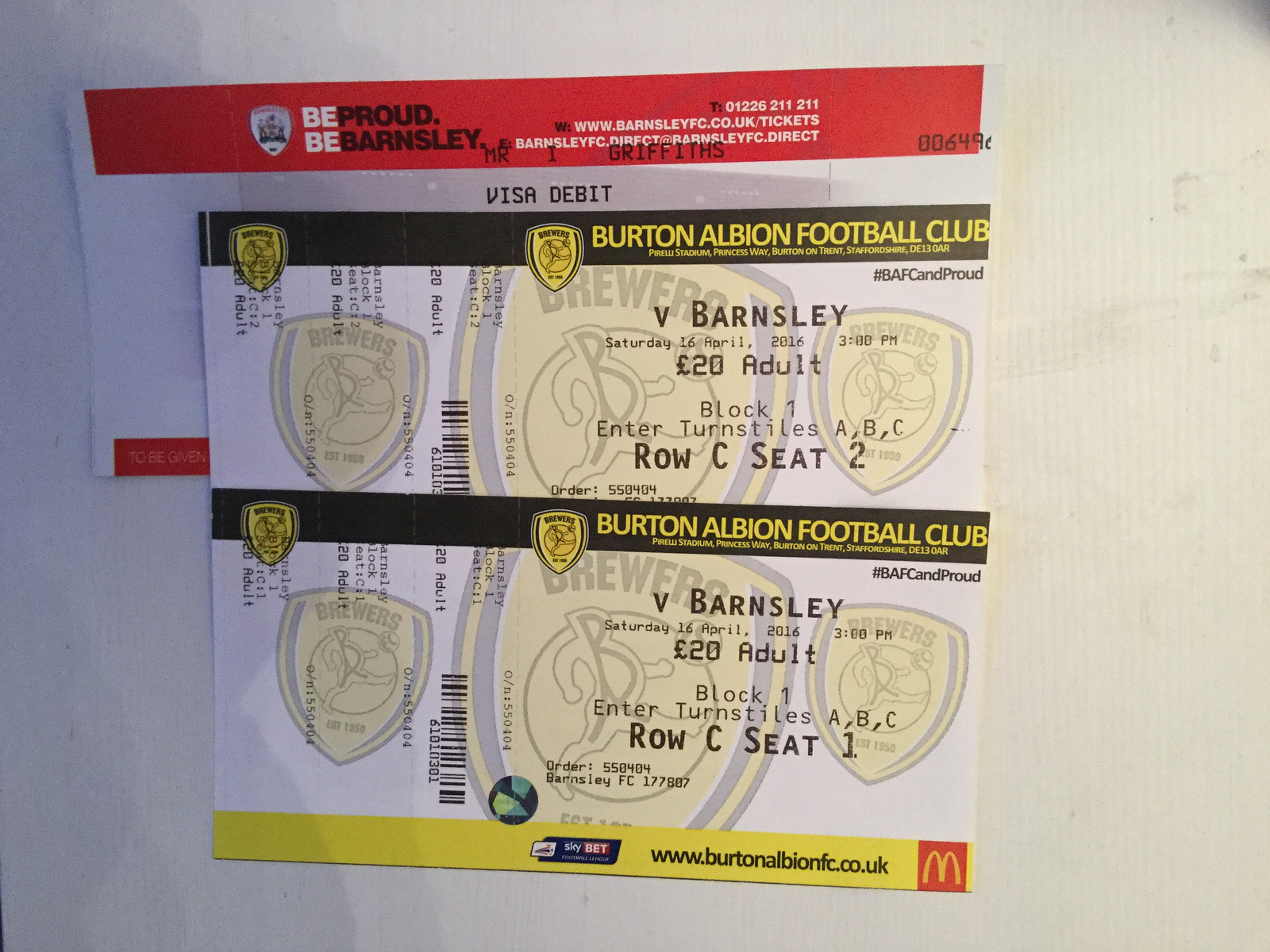The image showcases two unused tickets for a Burton Albion Football Club match against Barnsley, set on a white backdrop. Both tickets, printed with a black stripe at the top and a yellow stripe at the bottom, include medallions and logos along with the match details: Saturday, 16th April 2016, 3:00 PM. Each ticket, priced at $20 for adults, is for Block 1, with seat assignments being Seat 1 and Seat 2 in Row C, respectively. The tickets feature a barcode for entry through Turnstile A. Prominent on the yellow stripe are a SkyBet advertisement, McDonald's logo, and an email address. Positioned beneath the tickets is a partially visible receipt or Visa Debit slip, hinting at their recent purchase.